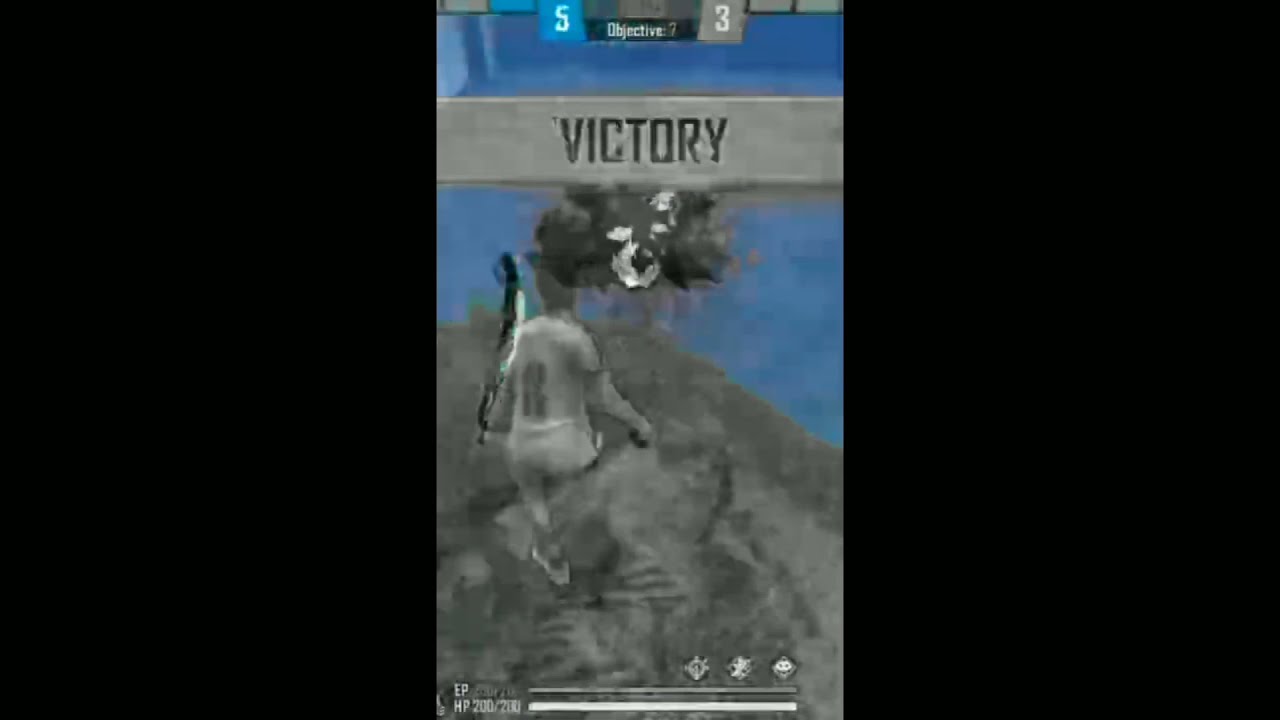This image appears to be a screenshot from a mobile video game, featuring a victory screen. The center third of the image contains the game-related elements, while the left and right thirds are large black bars. At the top, there is a grey bar with etched writing, reading "Victory." Just above this bar, the score is displayed: a blue "5" on the left and a grey "3" on the right. 

The image is highly pixelated and grainy, making details hard to discern. In the middle of the screen, there appears to be a figure running on what looks like a large grey structure, possibly a mountainside or a rock. This figure wears a white jersey with the number "8" and matching white pants, and might be holding a black object, which is unclear due to the pixelation.

Underneath the figure, there is a health bar alongside other game metrics that are nearly indiscernible due to the poor resolution. The overall coloration in the scene involves shades of grey and hints of blue, adding to the sense of a blurred, heavily distorted visual, typical of zoomed-in, low-resolution images.